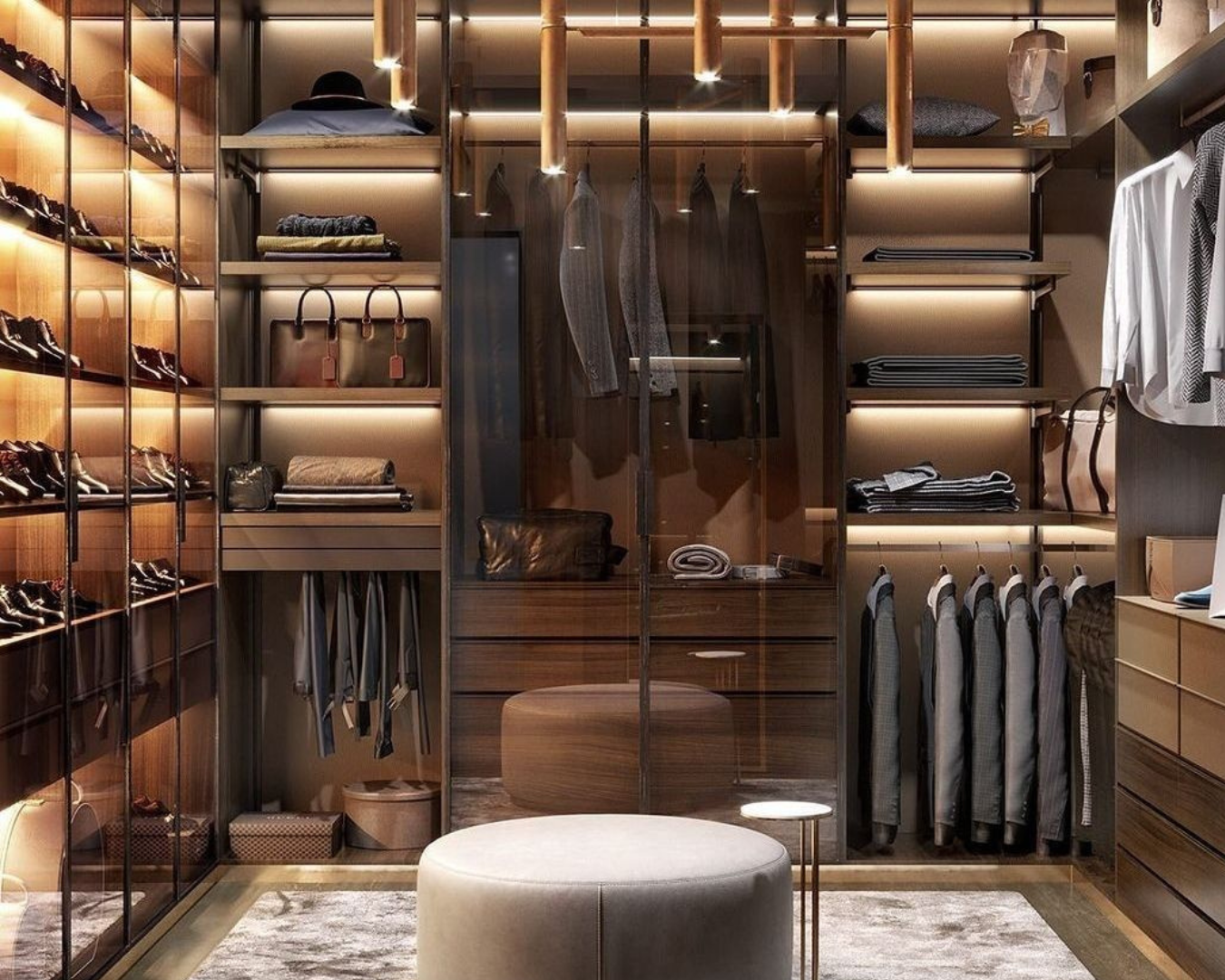The image is a detailed 3D color illustration rendering of an opulent men's suit store that resembles a lavish walk-in closet, possibly created using a design app like SketchUp. The store features a central round beige ottoman placed atop an abstract cream-colored rug, providing a chic seating area. The back wall boasts a set of glass doors, with the upper portion adorned by a hanging rack displaying an array of neatly arranged jackets. Below it, there are additional shelves holding various objects.

On the right side, the setup includes a top section dedicated to hanging shirts, complete with basket storage above and multiple shelves below, including pull-out drawers in a mix of beige and dark brown tones. The left side is primarily shoe storage, with numerous pairs of shoes meticulously placed on each shelf behind clear glass windows and doors. There are also purses, folded pants, and other items on the left side.

The entire space is illuminated by designer lighting from the ceiling, enhancing the luxurious atmosphere. The high-quality, well-organized displays suggest it is a high-priced, premium store catering to men, offering not just suits and pants, but also leather shoes, belts, bags, and even hats. Each section of the store is specifically designated: one for blazers and coats, one for shirts, another for handbags and boots, and a glass-covered area for additional high-end items. This sophisticated and meticulously designed interior is indeed the place to go for a high-quality, tailored shopping experience.